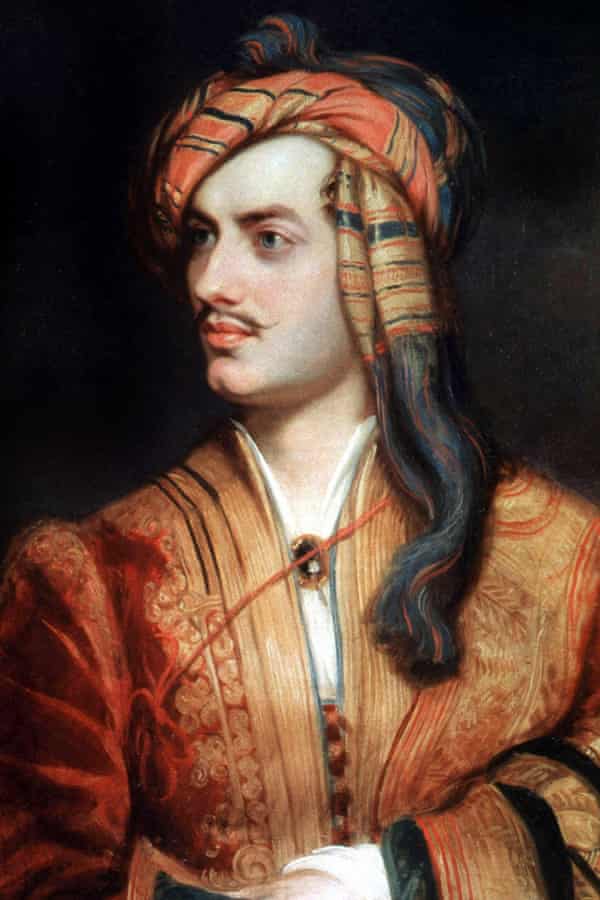The painting depicts a white man from an earlier era, centered and visible from the torso up. He has distinctive blue eyes, pronounced eyebrows, and a pencil-thin mustache above his pink lips. A notable feature of his face is a slight cleft chin. The man is looking off to his right with his left arm crossed in front of his chest, the right arm seemingly obscured or resting by his side. His attire is striking—a detailed, orangey-red suit with yellow trimmings and black strips on the sleeves, paired with a white undershirt peeking through the sleeves and beneath the jacket. A vivid scarf is wrapped around his head, predominantly red, yellow, and black, with the tail draping down the left side of his face. Around his neck, he wears a necklace with a gold and black center, possibly a brooch or a jewel, adding an element of ornate detail. The painting's background is dark, which accentuates the rich colors and intricate details of his clothing and accessories.